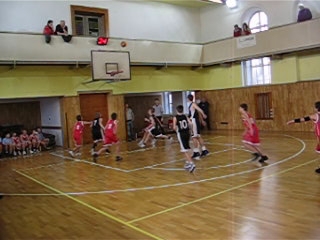This indoor color photograph captures a lively basketball game taking place in a gymnasium. The image is taken courtside, focusing on a cluster of young players, likely aged between 13 and 14, competing in front of one of the basketball hoops. The court features a light brown hardwood floor, marked with white lines delineating the playing area. 

In the center of the frame, a player in a blue jersey with a white number stands out prominently. Surrounding this central player are teammates in matching blue jerseys and opponents in red jerseys. On the left side of the image, there is a basketball backboard, and seated nearby on a bench are other players waiting for their turn to play.

In the background, the gymnasium's upper mezzanine or balcony is visible, resembling white walls and featuring several spectators who are intently watching the game. The balcony is accessed via a double doorway on the upper left side of the photograph. On the upper right, a window lets in bright natural light, adding to the overall clarity despite the slight blur in the image.